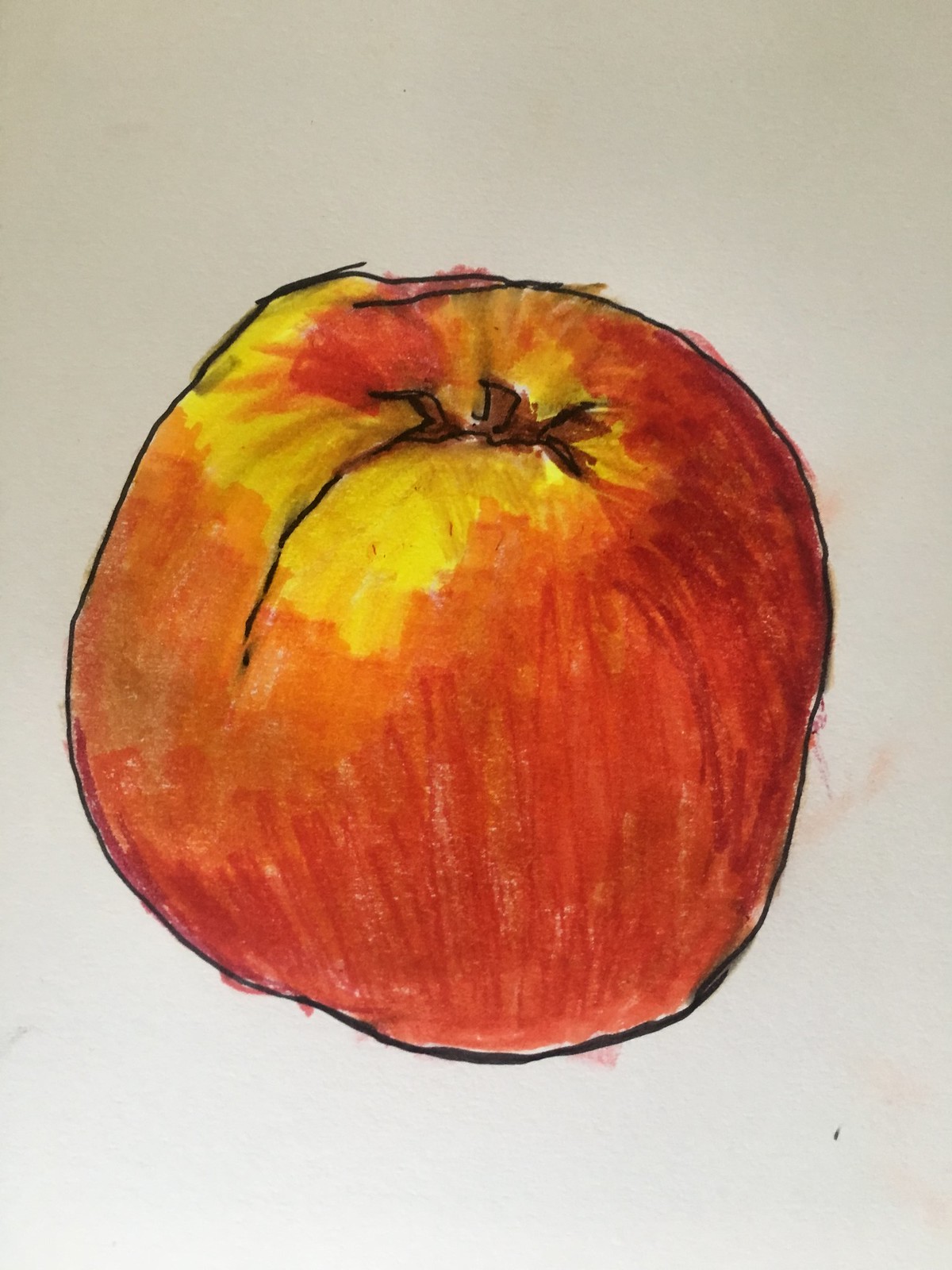The image features a piece of artwork that appears to be a blend of sketching and painting. The background is a tan-orange hue, providing a warm and neutral backdrop. Dominating the center of the composition is a depiction of a peach, characterized by its slightly irregular, circular shape. The peach is outlined in what seems to be ink, with its interior painted in vibrant shades of orange. Touches of yellow are strategically placed around the top and in a few other spots for added emphasis. The overall effect is a striking yet simple portrayal of the fruit against a minimalist background.